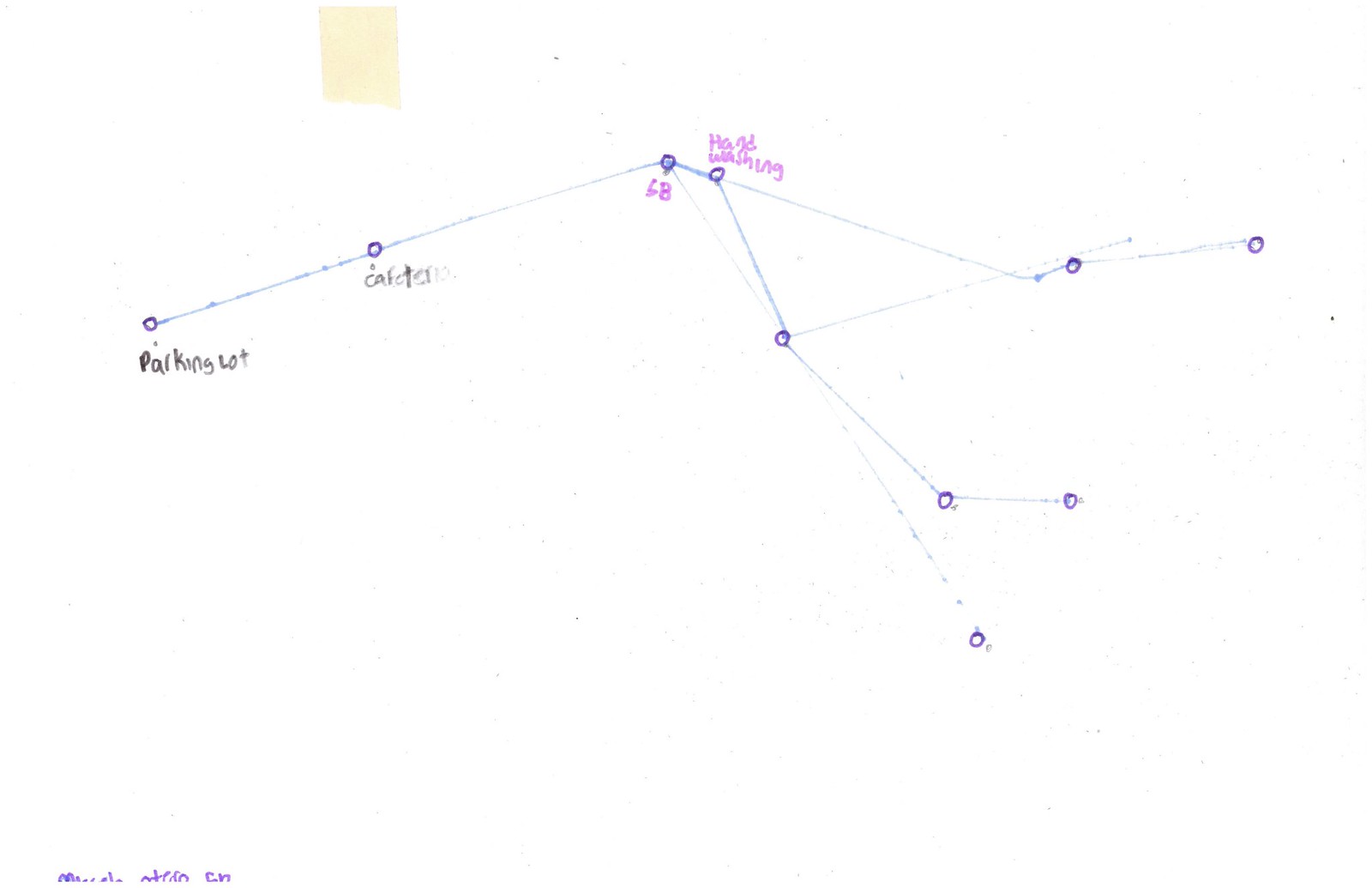The image appears to be a hand-drawn map featuring several key landmarks and directional lines in blue ink, likely drawn with a ruler for precision. 

On the far left side of the map, there is a label that reads "parking lot." From this point, a straight blue line extends upward and to the right towards the "cafeteria." Continuing further up and to the right, there's a marking labeled with the number "68." The line then descends diagonally to a dot labeled "housewashing." Beyond this, the map features additional blue lines forming a triangle before extending off to the right. 

There are more lines that travel downward and then bifurcate to the right. Notably, in the top-left corner of the map, there is a yellow square, which looks aged or perhaps as though it was left over from a previous iteration of the map. Additionally, there is some minuscule writing in the bottom-left corner, though it is too small to be legible. 

Overall, the map seems to serve as a guide to help locate various points of interest in a specific area.